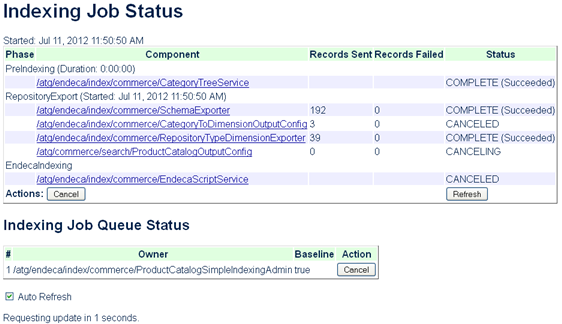In the image, we see an interface resembling an index file or status page. At the top, in bold black text on a white background, the title "Indexing Job Status" is clearly displayed. Just beneath that title, a date stamp reads "Started July 11, 2012, 11:50 AM," indicating when the indexing process initiated. 

Below the date stamp, a green header bar offers several menu options categorized under the headings: "Phase," "Component," "Records Sent," "Records Failed," and "Status." 

Under these headers, there are listed entries beginning with "Category Tree Service" followed by "Shima Explorer," "Category to Diminish Output Configuration," "Repository Type Dimension Exporter," and "Product Catalog Output Configuration." Additionally noted is "Indica Script Service." 

At the foot of the interface, two buttons are visible: a "Cancel" button and a "Refresh" button, presumably providing user interaction capabilities to manage the indexing process. The list entries suggest a detailed breakdown of components and phases involved in the indexing task, providing a comprehensive snapshot of its current progress and statuses.